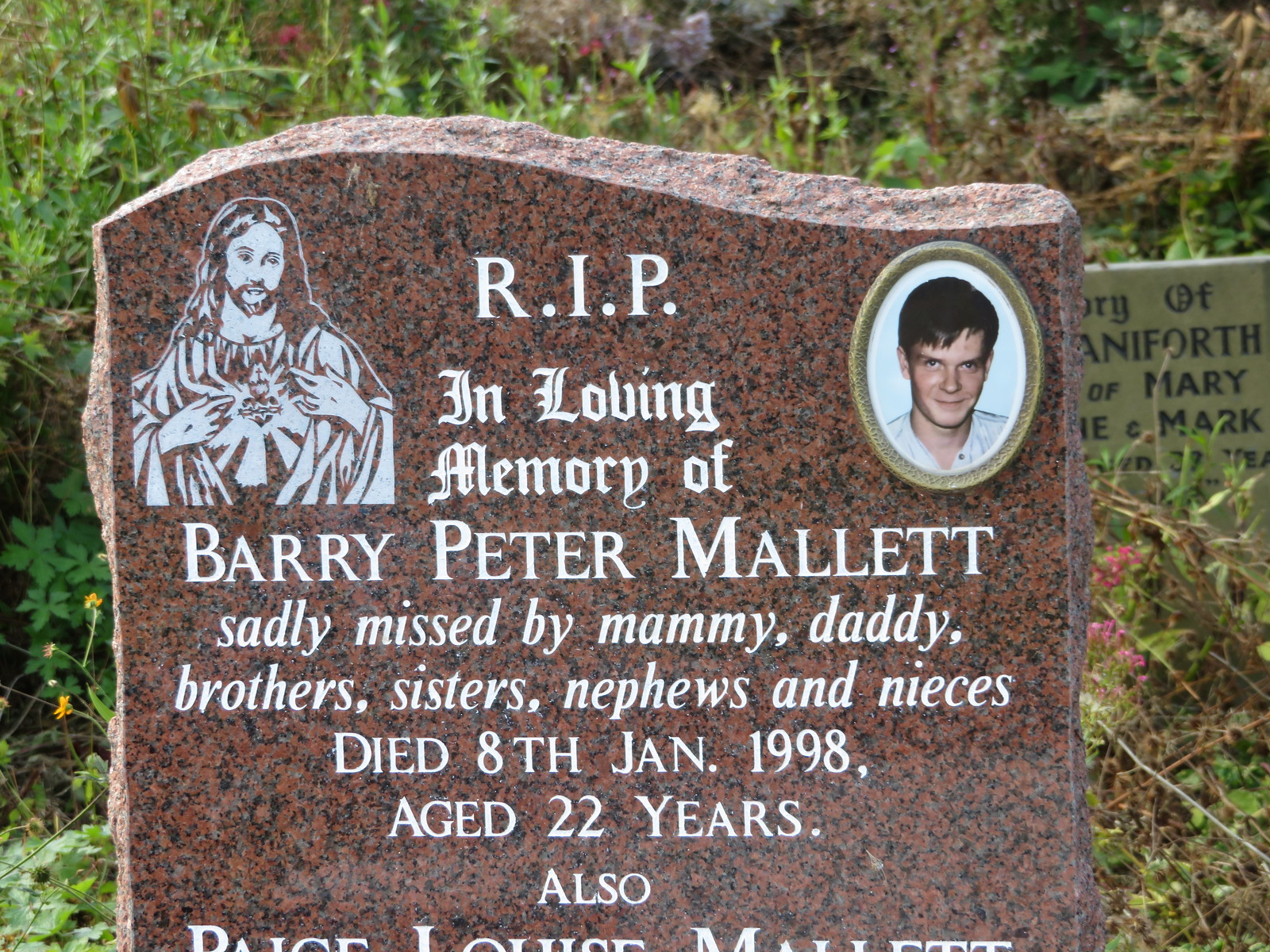This outdoor photograph, taken in a grassy area, captures a brownish-red marble tombstone dedicated to Barry Peter Mallett. The epitaph on the gravestone reads: "R.I.P. In loving memory of Barry Peter Mallett, sadly missed by mommy, daddy, brothers, sisters, nephews, and nieces. Died 8th January 1998, aged 22 years." The lower portion of the inscription is cut off by the photograph. In the top right corner of the tombstone is a round photograph of Barry, smiling in a white shirt, showcasing his short brown hair. To the left of the tombstone is a white engraving of Jesus with a glowing heart in the center. The background features overgrown vegetation and another tombstone to the right, partially visible and mentioning names Mary and Mark.